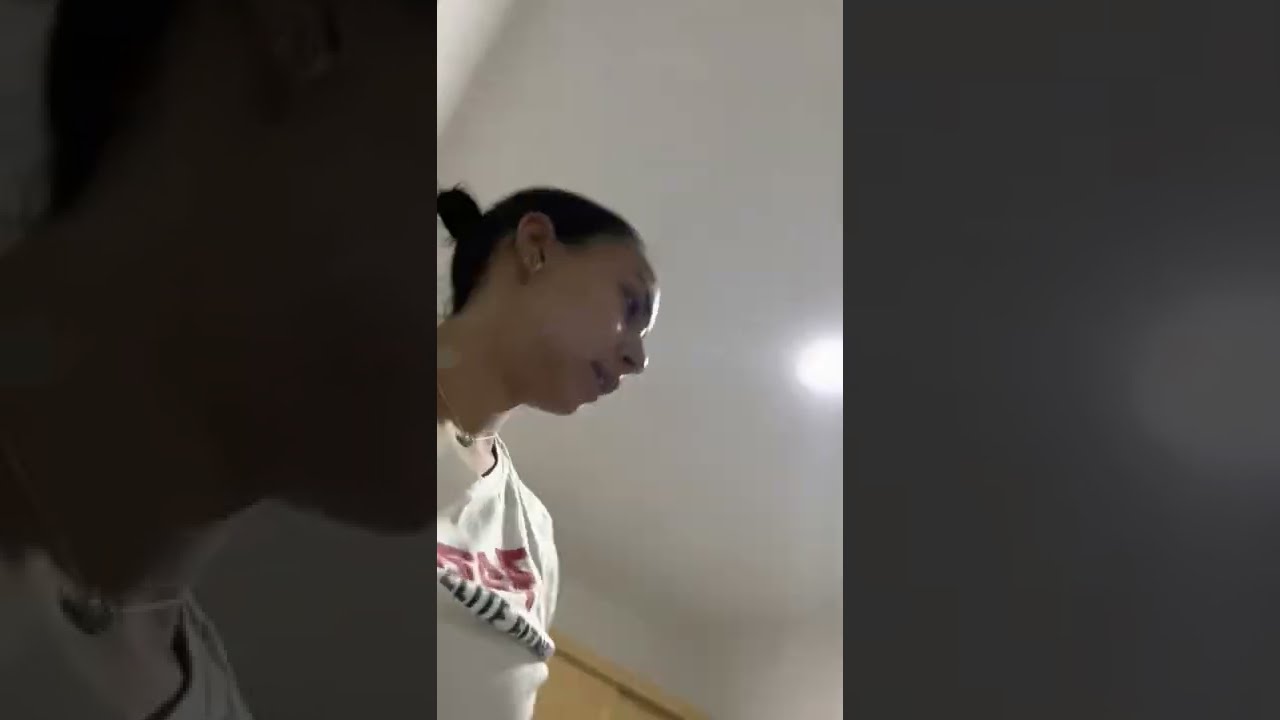The full-color photograph is a horizontally rectangular image composed of three vertically rectangular panels. The center panel is the smallest and the brightest, featuring a woman with dark hair pulled up in a bun and darker-colored skin, possibly brown. She is wearing earring studs and a white, short-sleeve t-shirt with red and black lettering that is partially obscured due to the shirt being bunched up. The black text appears to say "cliff fitness" or possibly "elite fitness," though it is not entirely clear. The woman is situated more towards the left side of the center panel, looking to the right, and appears to be in mid-conversation. There is a white light shining towards the right portion of the photograph, highlighting the scene. The left and right panels are darker and serve as blown-up, fragmented versions of the center panel, with the left close-up focusing on the woman and the right on the light. The background includes white walls, a white ceiling, a brown border on the wall, and a light wood-colored shelf. The woman has no discernible facial expression beyond her focused gaze.